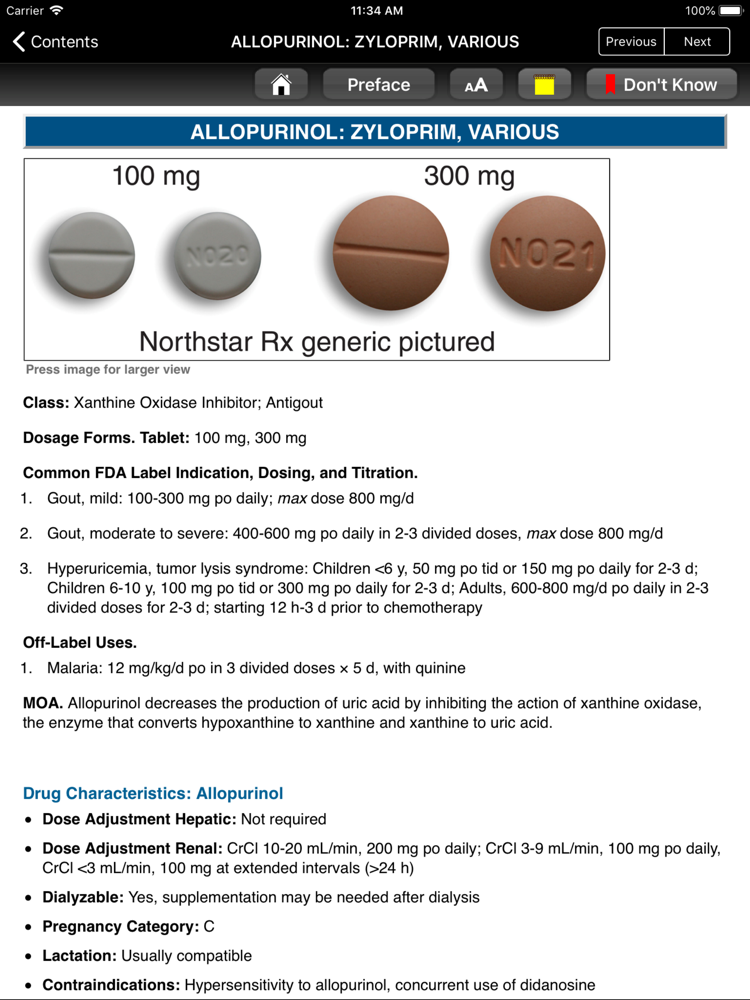Vertically oriented, the screenshot captures a cell phone display. At the top, a black horizontal banner features the following from left to right: the text 'Carrier', a Wi-Fi icon, the time '11:34 AM', the battery percentage '100%', and a battery icon. Below 'Carrier' on the left is a white back button accompanied by the main content in the center reading 'Allopurinol, Xyloprim, Various.' On the right side are 'Previous' and 'Next' buttons.

A dark blue horizontal banner situated underneath repeats the text 'Allopurinol, Xyloprim, Various.' Following this, there's a thin, black-outlined horizontal rectangle containing images of two different pills—100 mg and 300 mg. Each pill is depicted with both front and back views. Below these images, a label reads 'North Star RX Generic Pictured.'

The lower section of the screenshot provides detailed information about the medication, including class, dosage forms, common FDA label indication, dosing and titration, off-label uses, mechanism of action (MOA), and several drug characteristics: dose adjustment (hepatic), dose adjustment (renal), dialyzable status, pregnancy category, lactation considerations, and contraindications.